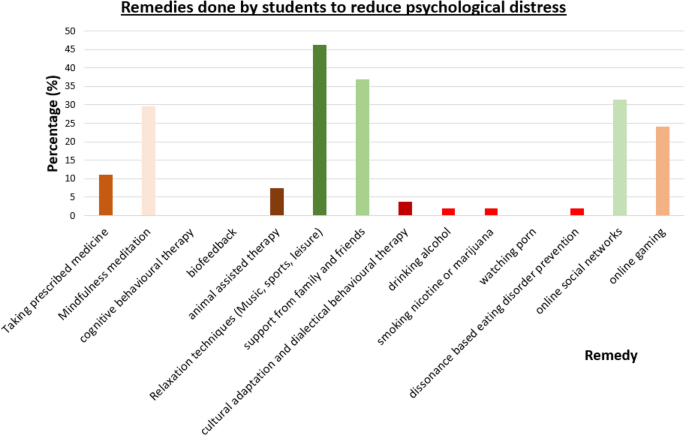This color bar chart titled "Remedies Done by Students to Reduce Psychological Distress" illustrates various techniques students employ to mitigate psychological distress, displayed with vividly colored bars. The y-axis enumerates remedies such as taking prescribed medicine, mindfulness meditation, cognitive behavioral therapy, biofeedback, animal-assisted therapy, relaxation techniques (including music, sports, and leisure), support from family and friends, cultural adaptation and dialectical behavior therapy, drinking alcohol, smoking nicotine or marijuana, watching porn, and engaging in dissonance-based eating disorder prevention. Additional remedies listed are engaging in online social networks and online gambling. The x-axis, marked in 5% increments from 0 to 50%, shows the percentage of students using each remedy, with horizontal lines aiding in readability. Most bars are shaded in varying hues of brown, tan, orange, red, and green. Notably, the highest reported remedy, relaxation techniques, reaches approximately 45%, while other remedies range from near 0% to around 35%. The chart is presented in black font with clear visual aids to enhance comprehension of the data distribution.